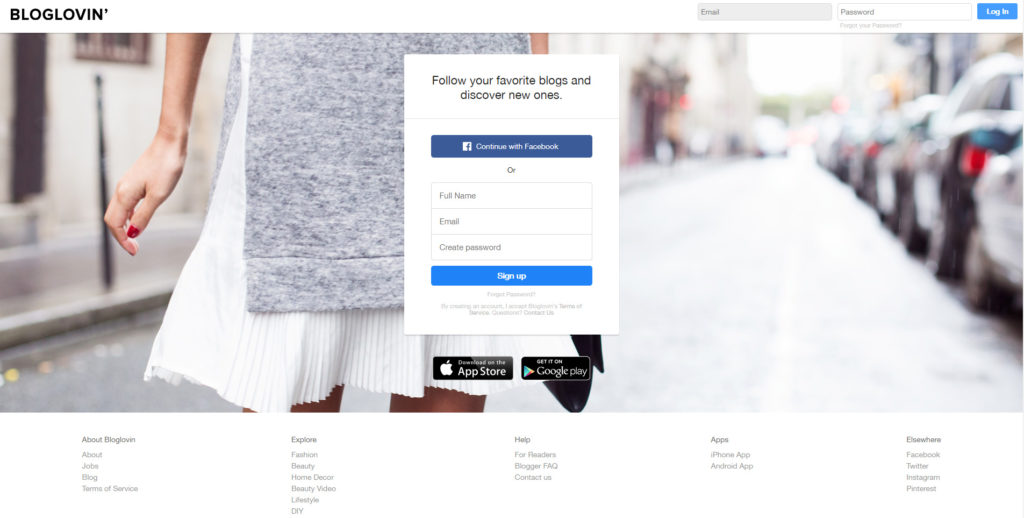This is a detailed screenshot of a webpage featuring the platform Bloglovin'. In the upper left corner, the site name "Bloglovin'" is prominently displayed, with an apostrophe replacing the 'g' in "loving." Directly to the right of the site name, there are fields for user credentials: an email field, a password field, and a Login button. Below the password field, a "Forgot your password?" hyperlink is provided for users needing assistance with their login details.